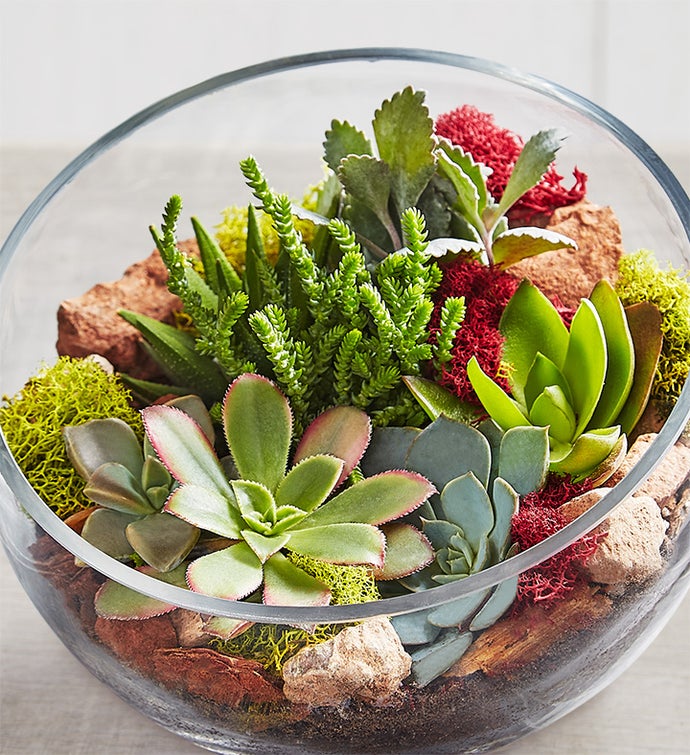This close-up photograph captures a meticulously crafted homemade terrarium housed in a simple glass bowl with gently curved edges. Inside this miniature botanical world, a variety of small cactus plants—ranging from light gray-green to deep green, lime, and even red—thrive, each displaying unique forms and hues. The base of the terrarium is covered in vibrant moss, featuring patches of red and green that add a rich, textured backdrop to the cacti. Scattered throughout the composition, an arrangement of stones in shades of white, red, and clay accents the design, primarily lining the outer edges of the bowl. The image offers an overhead perspective, inviting viewers to appreciate the intricate details and vibrant colors of this beautiful little plant display.